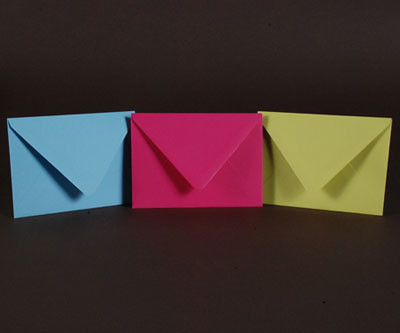The image features three vertically standing envelopes aligned horizontally against a solid black background. Each envelope displays its flap facing outward, slightly open. The left envelope is a bright, light blue, the middle one is a vibrant, deep pink bordering on magenta, and the right envelope is a muted yellow. The envelopes cast noticeable shadows on the background and on each other, with the pink envelope in the center slightly overlapping and casting shadows on the adjacent blue and yellow envelopes. The composition is simple, with a focus on the contrasting colors of the envelopes and their subtle interactions through shadow. The overall image is square in shape, and while not highly detailed, effectively highlights the primary colors of the envelopes against the stark black backdrop.